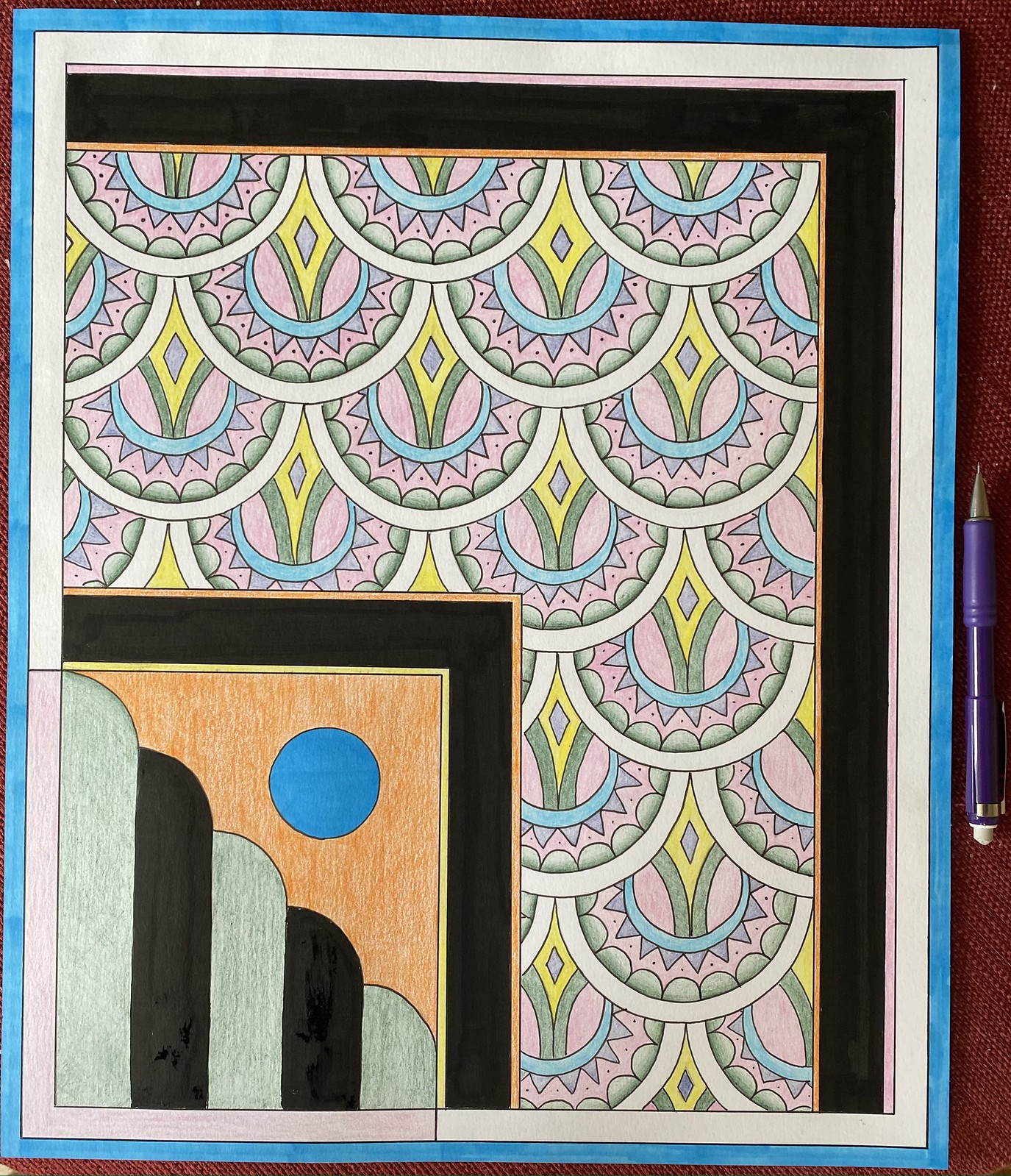This image appears to be a detailed piece of artwork set against a burgundy fabric background, with a purple ink pen placed to the right side. The artwork is vertically rectangular and framed with multiple layers: a light blue outer frame, followed by a white edge, then a pink edge, which transitions into a black margin, and finally into an orange edge. The central artwork features a vibrant, mosaic-like pattern composed of light blue, light green, white, pink, and yellow colors. The lower left corner of the artwork contains a distinct section: a square outlined in black, with layers transitioning from yellow to orange, incorporating a blue circle, and light green and black elements at the bottom. This section also includes overlapping rectangles of green and black with curved tops, set against a brown background with a blue circle above them and outlines of yellow, black, and brown. Additionally, there are oval-shaped pillars, varying in height and patterned in alternating gray and black, which are set against what appears to be petal-like shapes bordered with white and filled with small triangles. A central blue circle features a yellow diamond enclosing a gray center, contributing to the overall psychedelic and dynamic nature of the artwork.